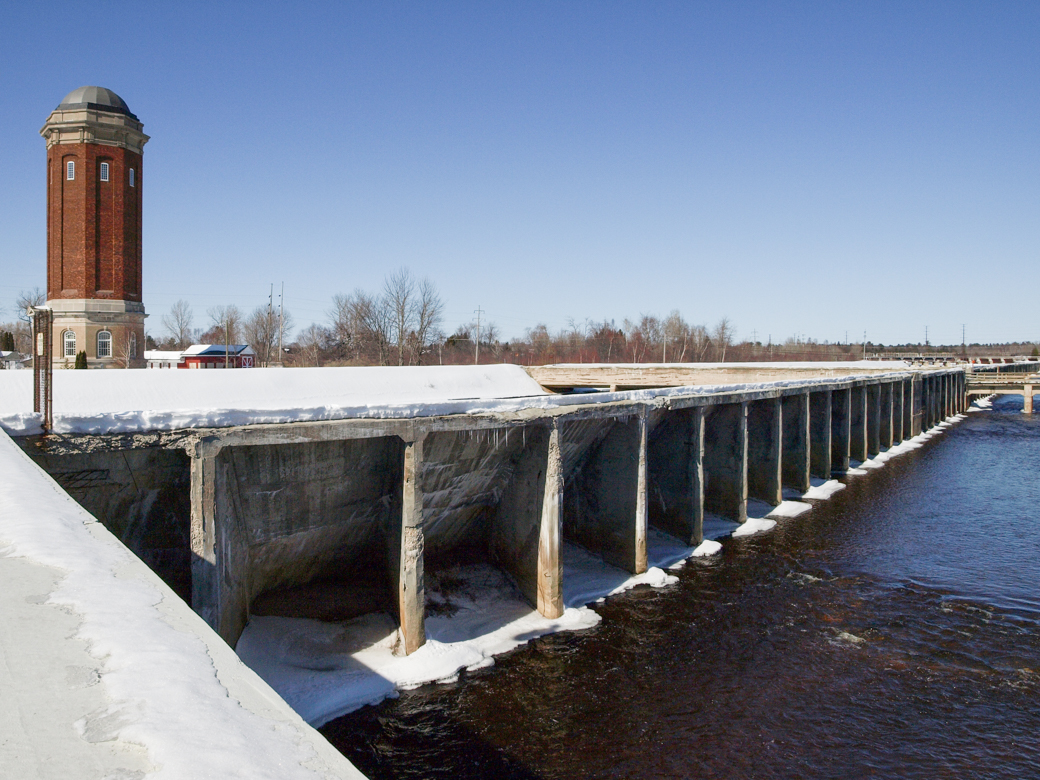This photograph captures a serene river scene dominated by a concrete dam structure, with no current water flow over its edge. You can observe the water flowing below the dam, appearing dark and murky. The sky is a clear, vibrant blue, suggesting a beautiful day. On the left side of the image stands a prominent brown tower, topped with either a gold or bronze dome, partially obscured by the dam itself. This tower seems to belong to a larger structure or building. The background is filled with leafless trees, indicating a winter setting, and there is a noticeable accumulation of snow atop the dam. Additionally, wooden pillars support a white-painted structure diagonally crossing the scene, possibly part of a bridge. The reflective quality of the water varies, with lighter blue hues near the top, mirroring the sky. The overall composition is devoid of any human or vehicle activity, emphasizing the stillness and tranquility of the area.